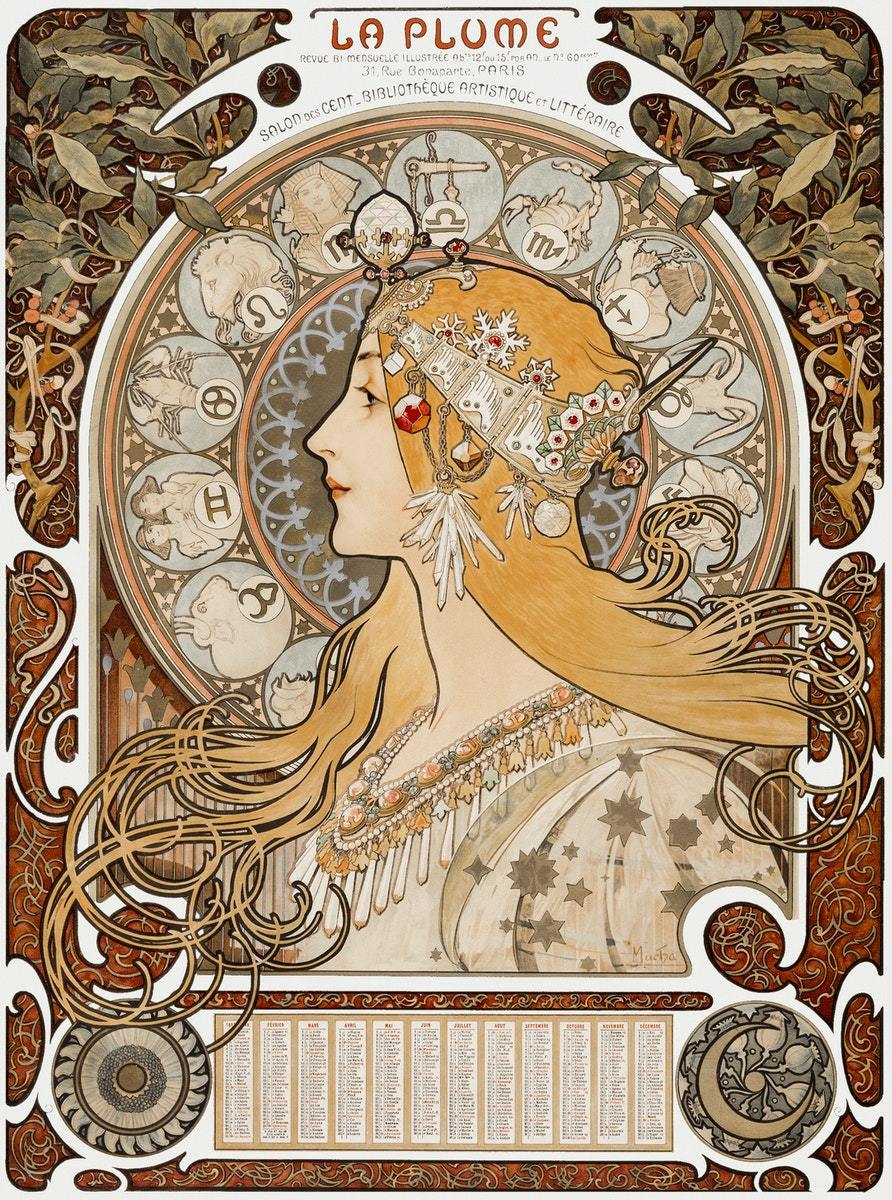The image is a vintage-style poster or flyer titled "La Plume" displayed in ornate, orange eccentric lettering at the top. Beneath the title, additional French text reads "Revue de Marseille, Illustré à venir 2 ou 5 mois" and "Salon d'Essence Bibliothèque Artistique et Littéraire." A central artistic element dominates the middle of the design featuring a side profile of a fair-skinned woman with long, curly blonde hair that ends in circular curls. She is depicted with orange lips and is gazing off to the left.

Adorning her head is an elaborate crown-like headband connected to her ears, embellished with gemstones, snowflake motifs, chains, feathers, and various jewels, with a horn-like protrusion in the front. Surrounding her head is a delicate halo comprised of different astrological zodiac signs, adding to the mystical and intricate detailing. The entire card is enriched with olive and beige tones, highlighted by muted olive leaves and vines that frame the top corners. Additional orange geometric patterns embellish the background, while at the bottom, small text is present along with illustrated symbols of the sun on the left and the moon on the right. The design exhibits extensive detail, crafting a regal and slightly ethereal visual appeal.